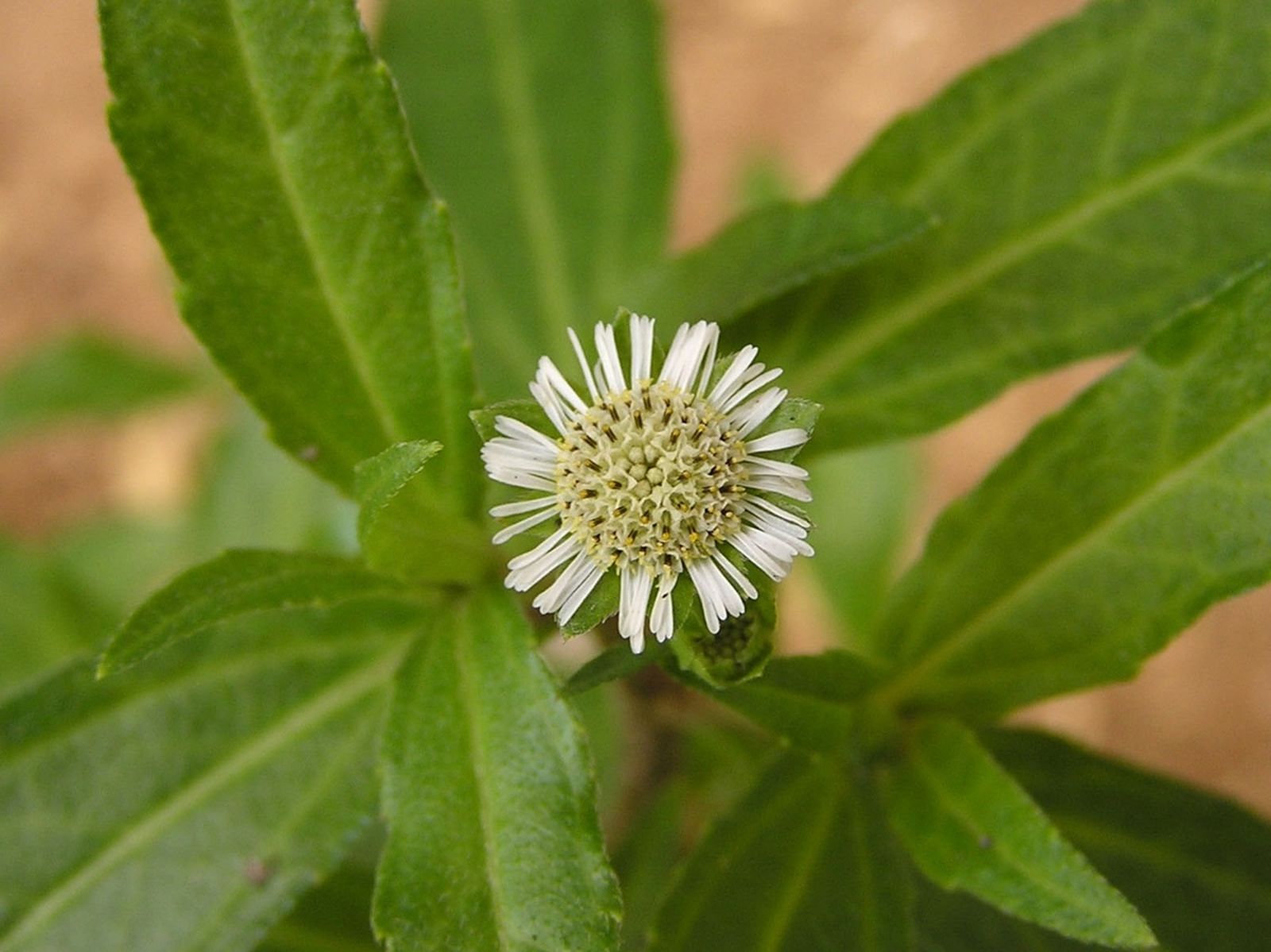The photograph showcases a meticulously detailed small flower at the center. The flower is characterized by its delicate, very thin, and white oblong-shaped petals, which sparsely encircle a prominent, yellowish-green central bulb resembling a round, half-spherical bud that contains various black and green filaments. The petals, although numerous, do not completely surround the bud, giving it an airy appearance. Surrounding the flower are several large green leaves with light green veins, distinct ridges, and pointed edges, all connected to a thicker green stem. The background is blurred with a tan hue, providing a contrast that emphasizes the green and white tones of the flower. The overall color palette of the image includes shades of green, white, off-yellow, and brown, which places the focus squarely on the intricate details of the small, delicate flower amidst its lush green foliage. This detailed depiction is likely part of a collection on plants and flowers, highlighting its botanical elegance.